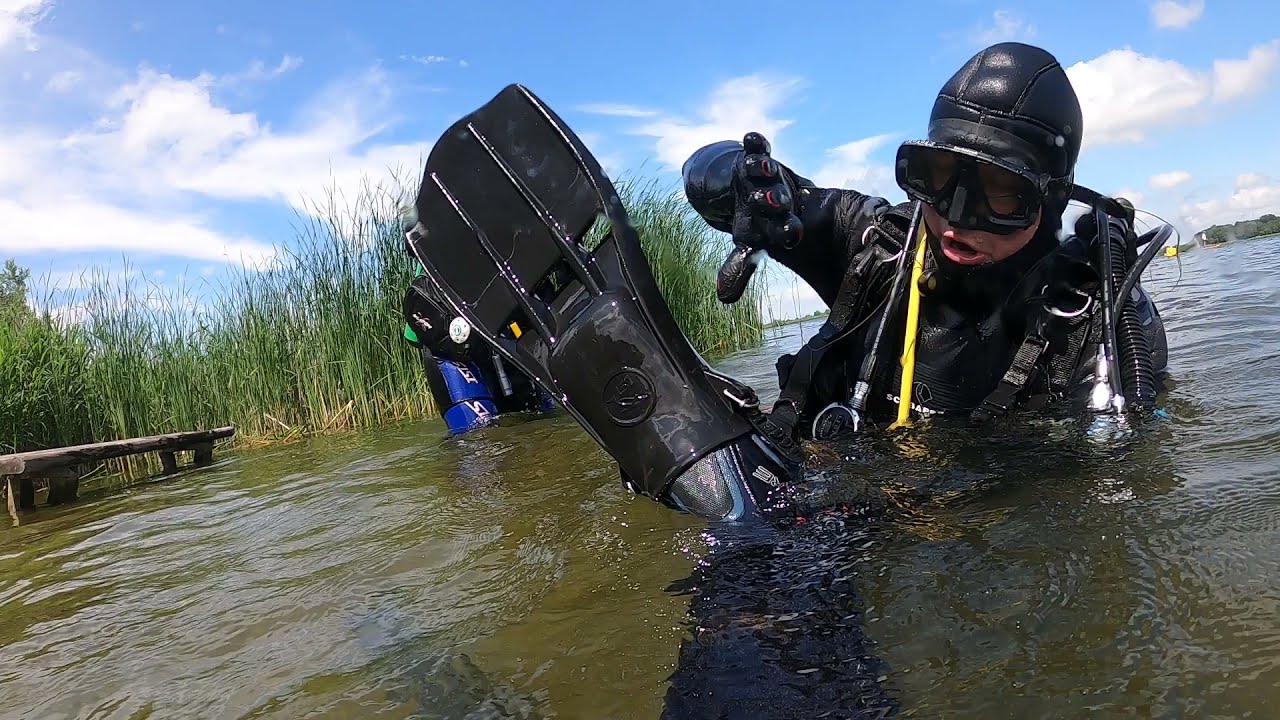The image displays a scuba diver emerging from shallow, murky, and muddy waters of a dark greenish earthy hue. The diver is clad entirely in black gear, including a wetsuit, gloved hands, black goggles, and a hood covering, with some yellow straps and tubing visible. The diver's mouth is open, and their hands are extended towards a large black flipper protruding from the water. Their face, partly visible, suggests they are Caucasian. In the background, tall green grasses and thin weeds peek out from the left side of the water, accompanied by a small wooden brown bench or piece of wood floating. The scene is set against a light blue sky dotted with puffy white clouds, and far off in the distance, a dock, a yellow object likely a boat, and possibly another person can be seen. The overall scene has a visible tilt towards the right, adding a dynamic touch to the composition.